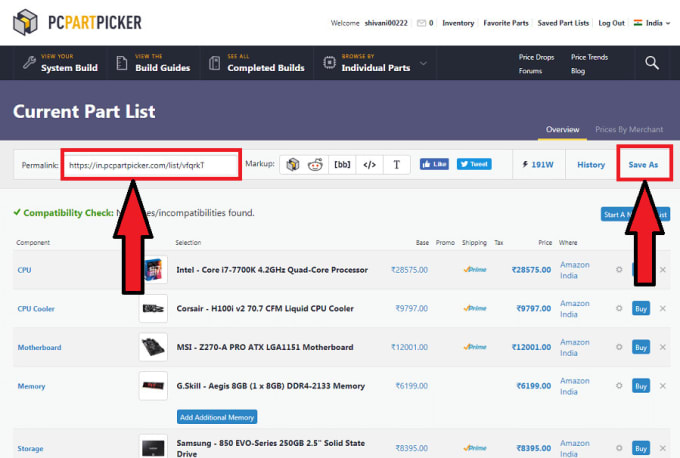This is a detailed screenshot of the "PC Part Picker" website. At the top, the header features the "PC Part Picker" logo alongside the site title in bold black and yellow letters set against a white background. Directly below, a black menu strip offers navigation options, including "System Build," "Build Guides," "Completed Builds," and "Individual Parts." On the far right of this strip, a search box is situated.

Beneath the menu, a blue header displays the "Current Part List" with two tabs: "Overview" and "Price by Merchant," with the "Overview" tab currently selected. Midway down the page, a permalink is highlighted within a red rectangular box, indicated by a red arrow. Similarly, another red arrow points to the "Save As" button, which also has a red rectangular box around it. The main section of the page showcases a comprehensive list of equipment and parts, allowing users to see the detailed components included in the current part list.